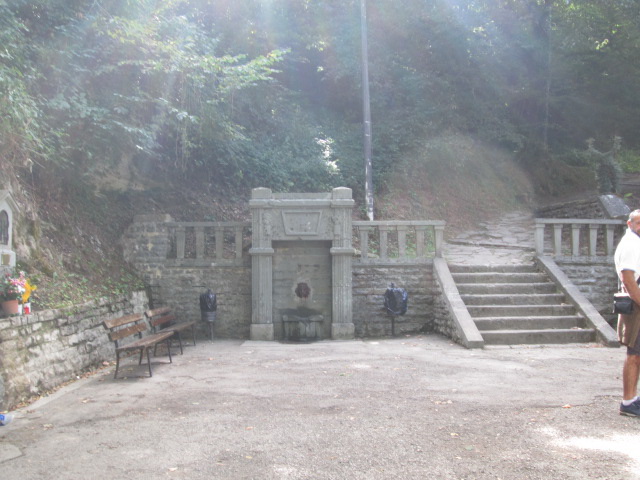The full-color outdoor daytime photograph captures a sunny scene in what seems to be a historic nature park or monument site. Sunlight streams warmly through the trees, creating visible rays and highlighting a small dust bubble often referred to as an "orb." Dominating the background is a stone staircase flanked by ancient architectural elements, possibly alluding to a small temple or monument. The staircase ascends a half-floor, hinting at an elevated area not entirely visible. To the left of the stone structure, two brown benches rest against a grayish brick wall, with flowers adding a touch of color to the setting. A well-maintained concrete plaza or walkway forms the foreground, where a man, presumably Caucasian, stands partially out of frame. He is dressed in a white shirt, brown or beige shorts, and carries a satchel. His head is partially cut off in the image, but his attire and stance suggest casual exploration. The lush, green foliage and numerous trees in the background accentuate the park's serene and historic ambiance.